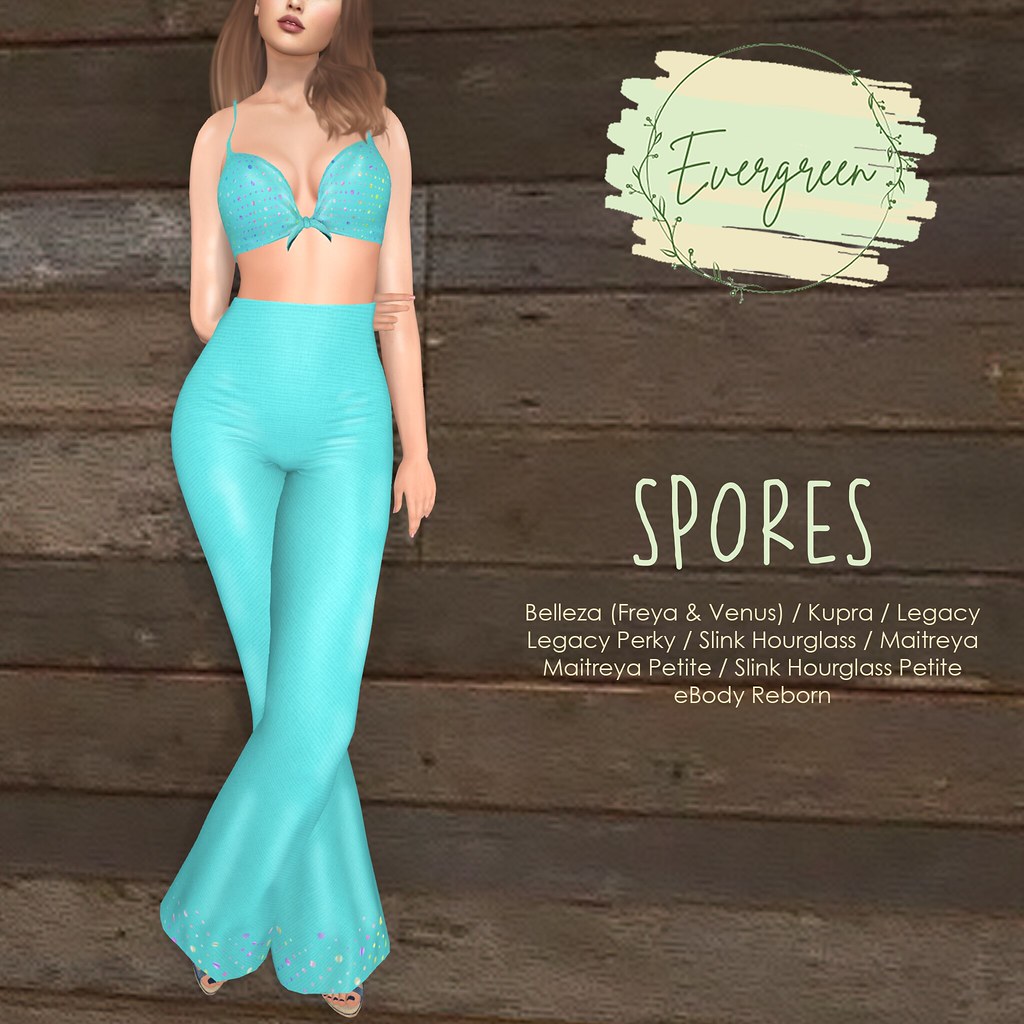The image depicts an advertisement set against a dark brown wooden plank background. On the left side stands a CGI model of a Caucasian woman with dark blonde hair that falls just below her shoulders. She is wearing a light teal or turquoise outfit comprising a swimsuit top and bell-bottom pants that reach down to her feet, obscuring any footwear. Her pose shows one arm wrapped behind her body, while her other hand rests on her waist. Her face is cropped, revealing only red lips and part of her nose.

On the upper right, there's a logo featuring the word "Evergreen" in cursive green letters encircled by a plant motif, displayed against a light patch of pink and blue paint that forms a makeshift rectangle. Just below this logo, in bold capital letters, is the word "Sporce." Beneath "Sporce," the following terms are listed in smaller font: Beleza Freya Venus, Cupra Legacy Legacy Perky, Slink Hourglass Maitreya Maitreya Petite, Slink Hourglass Petite, and Ebody Reborn.